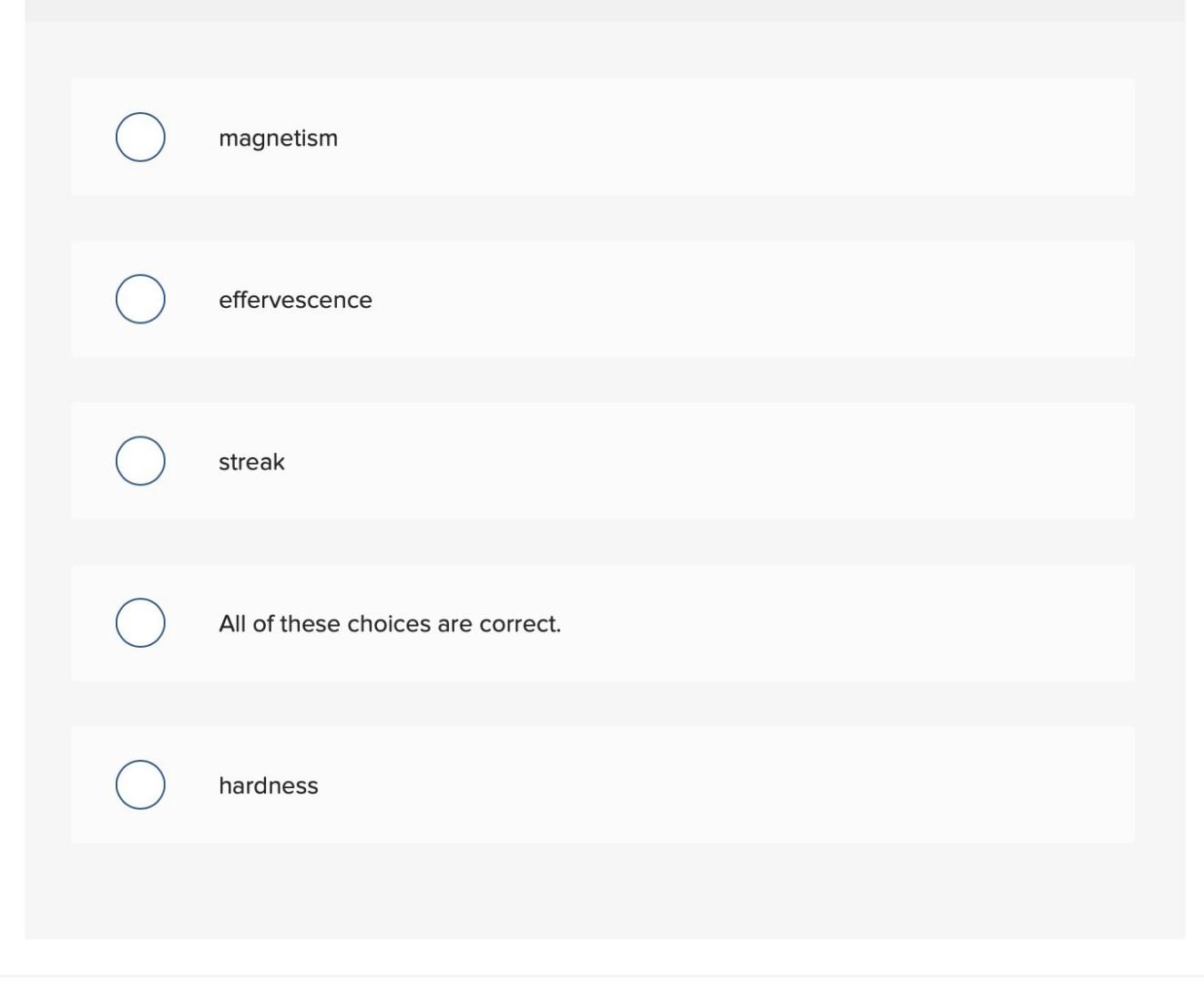A detailed caption for the image could be:

"This screenshot showcases a set of multiple-choice options, likely from a quiz or test. There are five distinct choices displayed in white horizontal bars, each accompanied by a circular selection indicator on the left. The choices listed are: 'Magnetism,' 'Effervescence,' 'Streak,' and 'Hardness,' with each option being marked as correct. The selection circles, filled with white, are either navy blue or black in color, contributing to a clear and organized visual presentation on a white background."